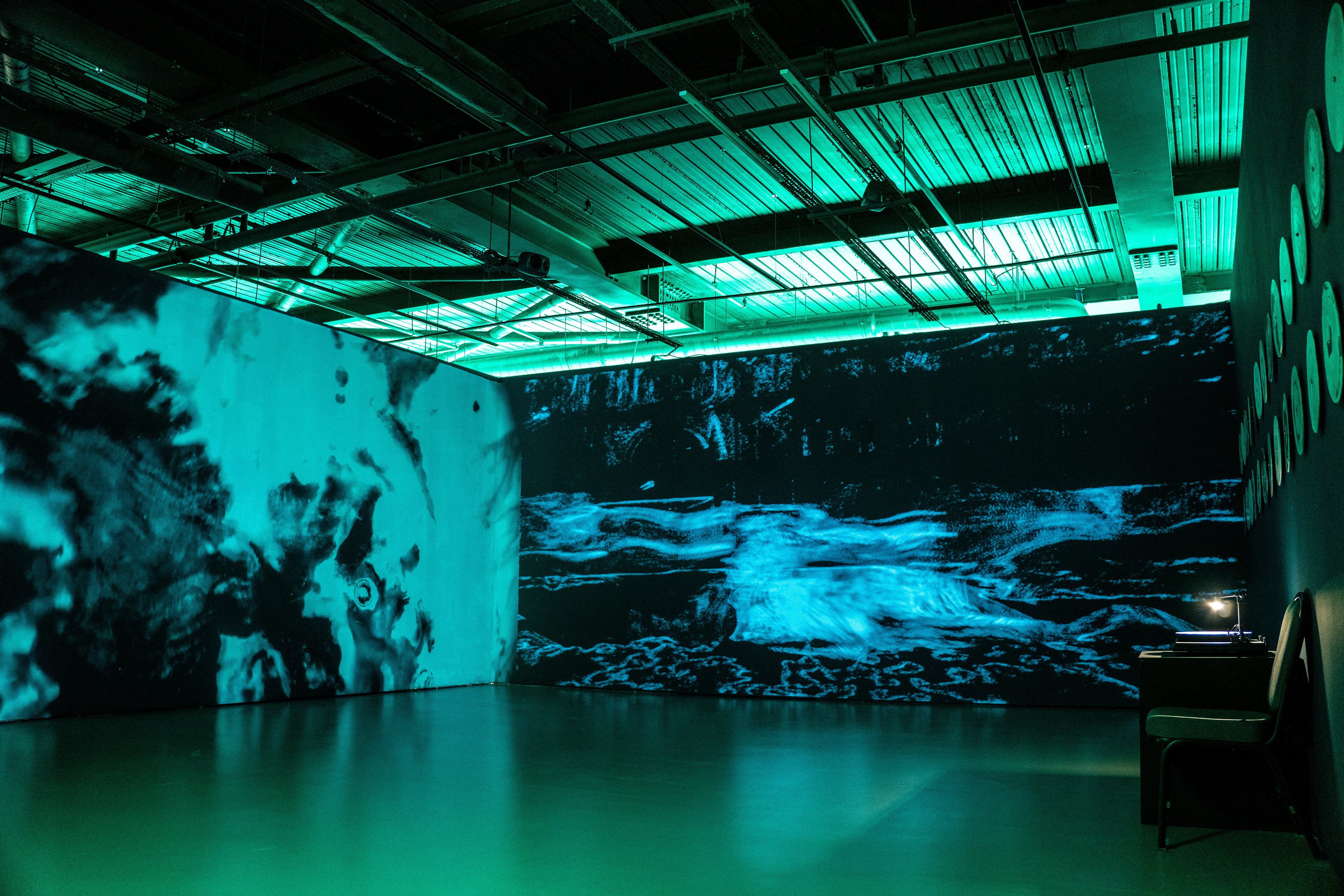The photograph depicts the interior of a spacious repurposed warehouse, now serving as an art studio or office space. The ceiling retains the typical industrial warehouse features with visible steel and iron railings, metal bars, aluminum roofing, and pipes running along it, adorned with lights and cameras, all bathed in a green hue from ambient lighting. The floor is notably flat and shiny, also displaying a greenish tint. The walls, which have been erected within the warehouse, feature psychedelic visual art comprising ink blob patterns, either painted directly or projected onto the black and light blue surfaces, illuminated by specialized lighting. Notably, the right wall is adorned with two rows of approximately 20 clocks. Below this array of timepieces, there is a desk and chair setup. On the desk, there is a projector or some machine casting light onto the wall, contributing to the room's artistic ambiance.